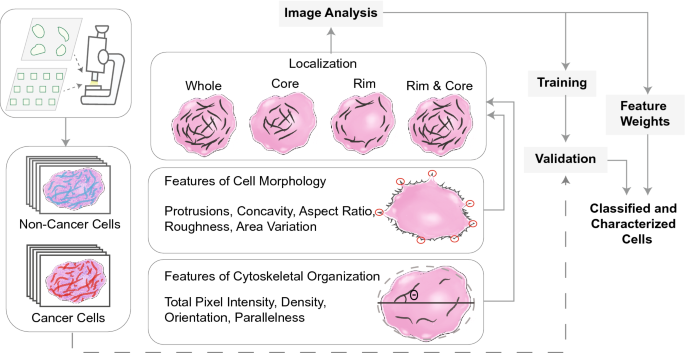An educational, multi-color digital image primarily themed around cancer analysis, set on a white background, comprises a detailed flowchart depicting various stages of image analysis in cell biology. The flowchart is titled "Image Analysis," and features black text throughout. 

In the upper left corner, there is an illustration of a microscope examining a yellow sample. Below the microscope are images of slides with cancer and non-cancer cells distinguished by color: non-cancer cells in pink with blue structures and cancer cells in pink with red structures. The central section of the image focuses on "Localization," showcasing four examples of cell localization: whole, core, rim, and rim and core, all in various pink shades and with black internal structures.

Further below, the diagram highlights "Features of Cell Morphology" including aspects such as protrusions, concavity, aspect ratio, roughness, and area variation, displayed through a pink cell with circled red spikes. Adjacent to it, "Features of Cytoskeletal Organization" are detailed, featuring aspects like total pixel intensity, density, orientation, and parallelness, with the cell illustrated in pink and black with a center division and fewer internal structures.

On the right side, the diagram transitions through the stages of "Training," "Feature Weights," "Validation," and culminates in "Classified and Characterized Cells." These stages are interconnected with arrows, clearly guiding the flow of the analysis process.